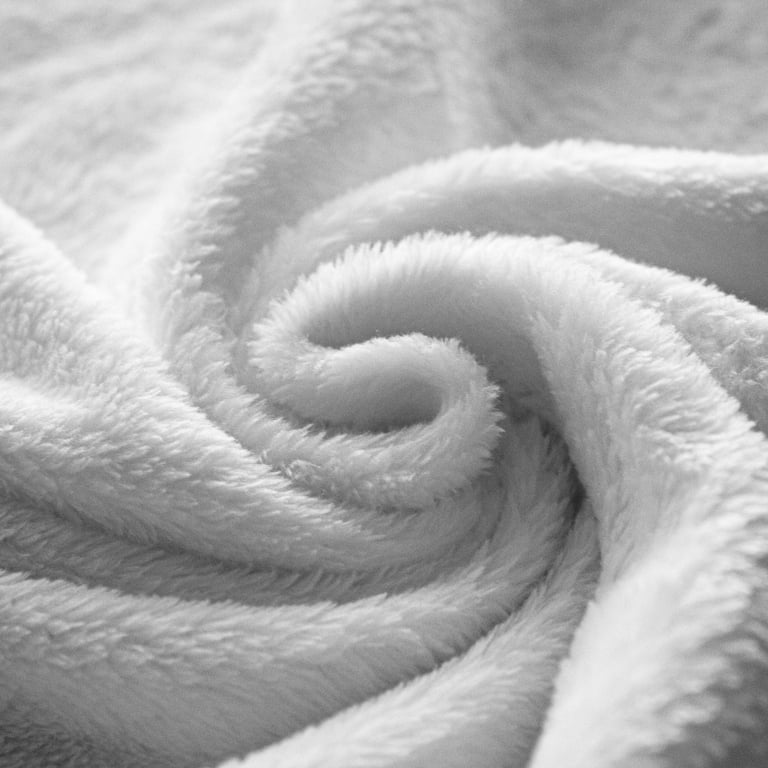This close-up image captures the intricate details of a pristine, white fabric, possibly a new blanket or fluffy towel. The texture is strikingly soft and luxurious, with fibers that stand upright rather than being matted down, indicating its fresh, unused state. At the center, the fabric is spun into a circular pattern, suggesting that someone pressed their pointer finger into the middle and twisted their fingers around, creating a clockwise swirl that radiates outward. Subtle shadows are cast across the fabric, hinting at the natural sunlight streaming in through a window, imbuing the scene with a warm, daytime ambiance. The close-up perspective and interplay of light and shadow emphasize the fabric's sumptuous texture and pure whiteness.